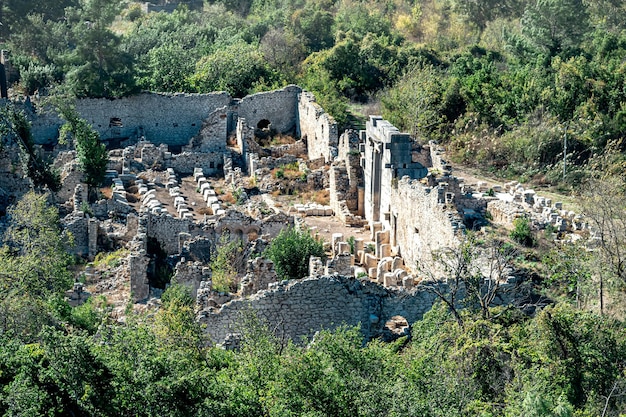This image provides an aerial or bird's eye view, seemingly captured from a hillside, of an ancient brick-walled ruin surrounded by dense greenery. The primary focus is a dilapidated structure in the center-left of the photo, characterized by its crumbling walls. One prominent wall extends from the left side, partitions halfway across the image, and runs parallel down towards the front before turning back to the left. Inside the structure, there are remnants of other walls that suggest it once housed multiple rooms or homes, now eroded and fallen over time.

Within the ruin, particularly in the upper left and bottom right sections, there are clusters of small stones which resemble gravestones, but are more likely fragments of the original building material. The entire site is enveloped by lush green trees and shrubs, adding to its secluded and ancient ambiance. Just outside the right of the ruin, a dirt road can be partially seen, bordered by more greenery and trees, though no clear access point to the structure is visible. This serene setting, combined with the deteriorated state of the ruins, indicates a long-abandoned site slowly being reclaimed by nature.